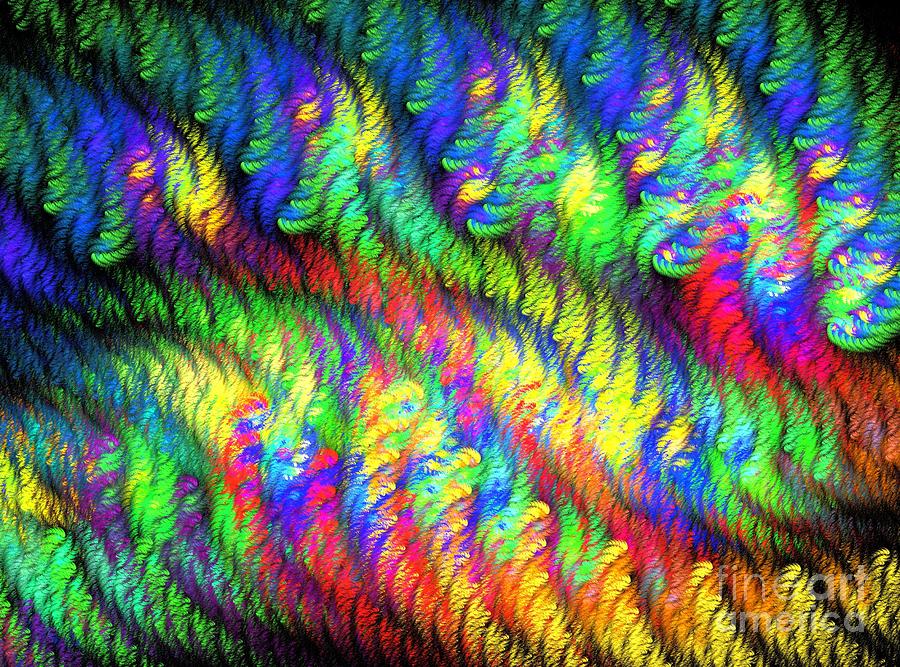This is a vibrant computerized artwork reminiscent of modern art or a digital drawing created in software like Photoshop or Illustrator. The composition features an elaborate, wavy pattern of intertwined colors, including blue, yellow, red, orange, purple, green, and black, set against a black background. The pattern starts with green at a corner and extends diagonally, becoming progressively tighter and more intricate in the lower middle with a blend of yellow, red, and blue hues. The design resembles bird feathers or a cable knit texture, with two distinct rows: the lower row is denser and the upper row more relaxed, appearing almost like a psychedelic tie-dye. Across the image, the colors weave seamlessly into each other, creating a visually captivating piece. In the lower right corner, there’s a faint white watermark reading "Fine Art America."